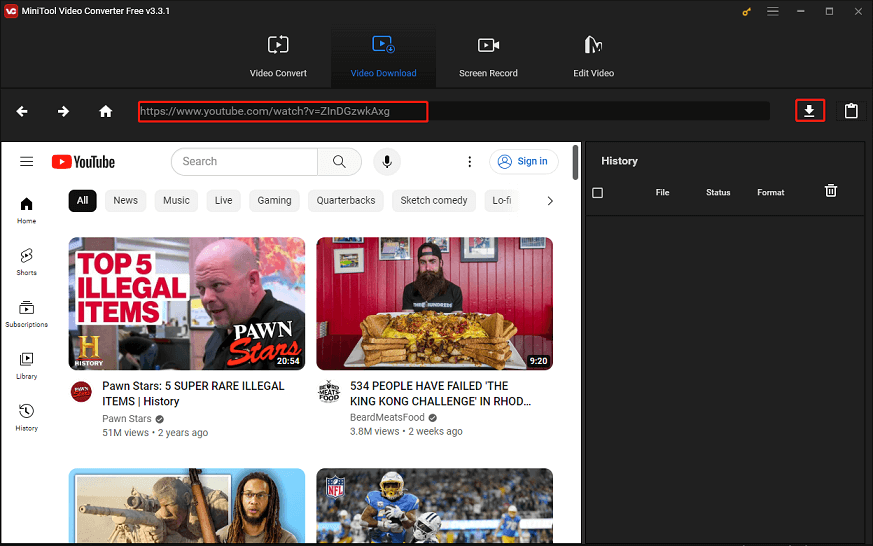This screenshot showcases the interface of a free video converter application. The background is predominantly black, allowing the various interface elements to stand out clearly. The cropped image prominently features the app's logo in small white font located at the top left corner.

At the top center of the screenshot, four large icons are arranged horizontally, each representing different functionalities of the app. The icons are labeled as follows: "Video Convert," "Video Download," "Screen Record," and "Exit Video." The "Video Download" option is highlighted in light blue, indicating it is currently selected.

Beneath these icons lies a search bar, highlighted with a red box around the text input area to emphasize where users should type the URL or search query. To the right of the search bar, a small line icon with a down arrow is also enclosed in a red box, signifying the download button.

In addition to these elements, the bottom left of the screenshot displays an overlaid window titled "Open YouTube Page," providing direct access within the app to YouTube's interface for easier video downloading. This visual composition is designed to make the app's functionality intuitive and user-friendly.